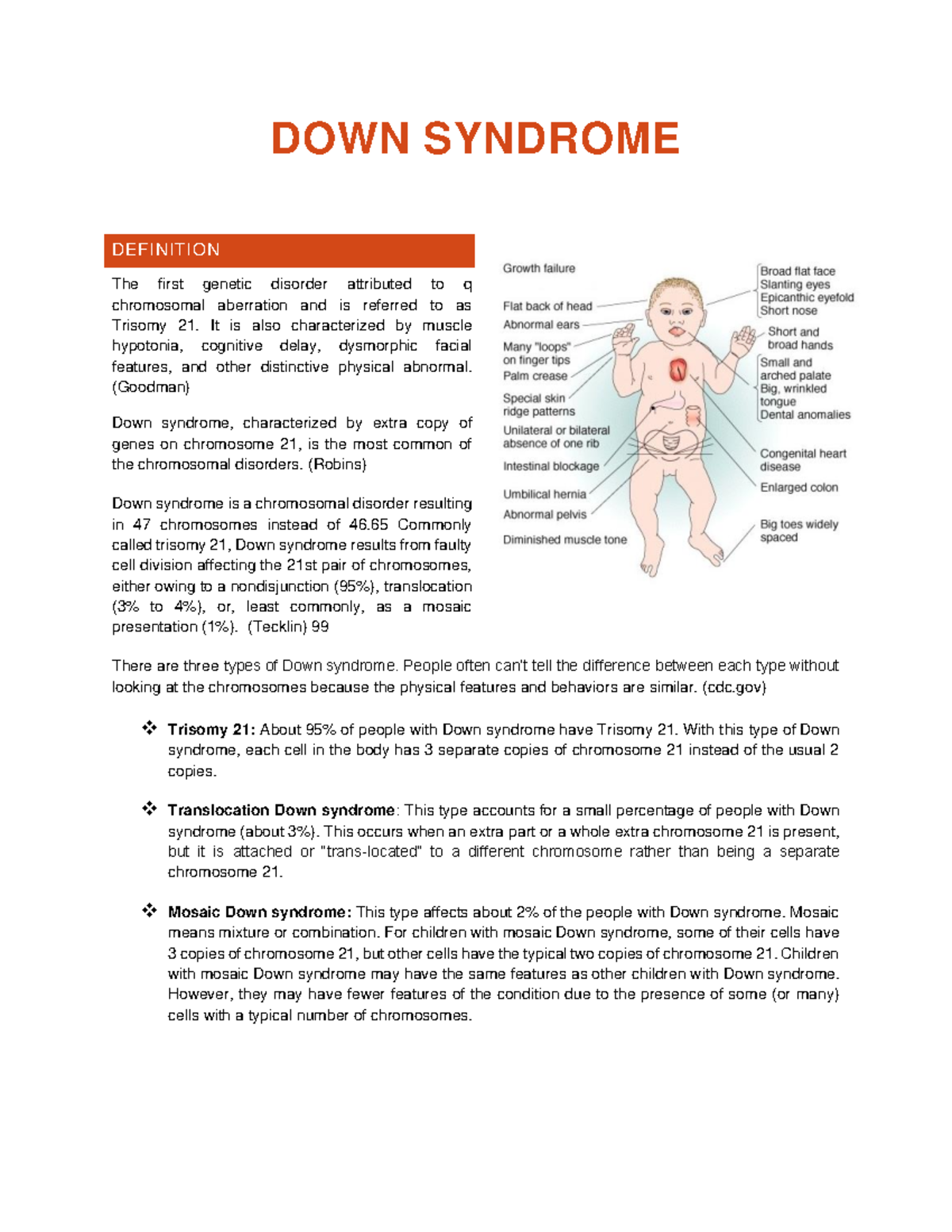The image is an educational display board typically found in a pediatrician's waiting room, providing detailed information about Down syndrome. The top section of the board features "DOWN SYNDROME" written in bold, red, uppercase letters. To the left, within a red rectangle, the word "Definition" is displayed in white font. Below, in black text, the definition reads: 

"Down syndrome is the first genetic disorder attributed to acute chromosomal aberration, specifically known as trisomy 21. It is characterized by muscle hypotonia, cognitive delay, dysmorphic facial features, and other distinctive physical abnormalities. This condition, resulting in an extra copy of genes on chromosome 21, is the most common chromosomal disorder."

Further down, the description elaborates:

"Down syndrome occurs when a person has 47 chromosomes instead of the typical 46. It commonly results from a faulty cell division affecting the 21st pair of chromosomes, due to non-disjunction, translocation, or, less commonly, a mosaic presentation. There are three types of Down syndrome:
1. Trisomy 21 - Present in about 95% of cases.
2. Translocation Down syndrome.
3. Mosaic Down syndrome - Present in about 2% of cases."

An image of a baby with blonde hair and fair skin is included to illustrate various symptoms. Labels point to specific features, indicating: 
- Big toes widely spaced, pointing at the toes 
- Congenital heart disease, pointing at the heart 
- Flat back of the head
- Growth failure
- Abnormal pelvis